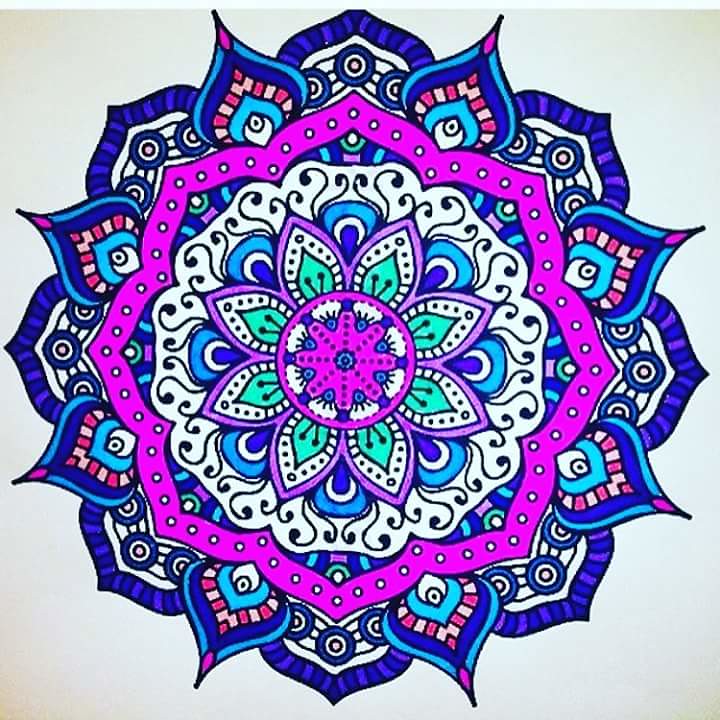A vibrantly colored mandala, reminiscent of a detailed coloring book page, dominates the image. At the center, a teal flower with a purple border graces the middle, accentuated by intricate twirly black lines extending outward. The central circle glows with hues of pink and purple. Encircling this core, dark blue petals emerge, highlighted by white rims and gradually transitioning into lighter shades of blue. Beyond this, a larger flower shape with a white background displays an elaborate pattern of black, vine-like designs. This section is enveloped by another flower-shaped layer, exhibiting a striking pink-magenta hue adorned with white dots. The outer rim of the mandala showcases a mesmerizing array of colors, including various shades of blue, indigo, and occasional touches of red and pink. The overall composition is a large, beautifully intricate flower-shaped mandala.